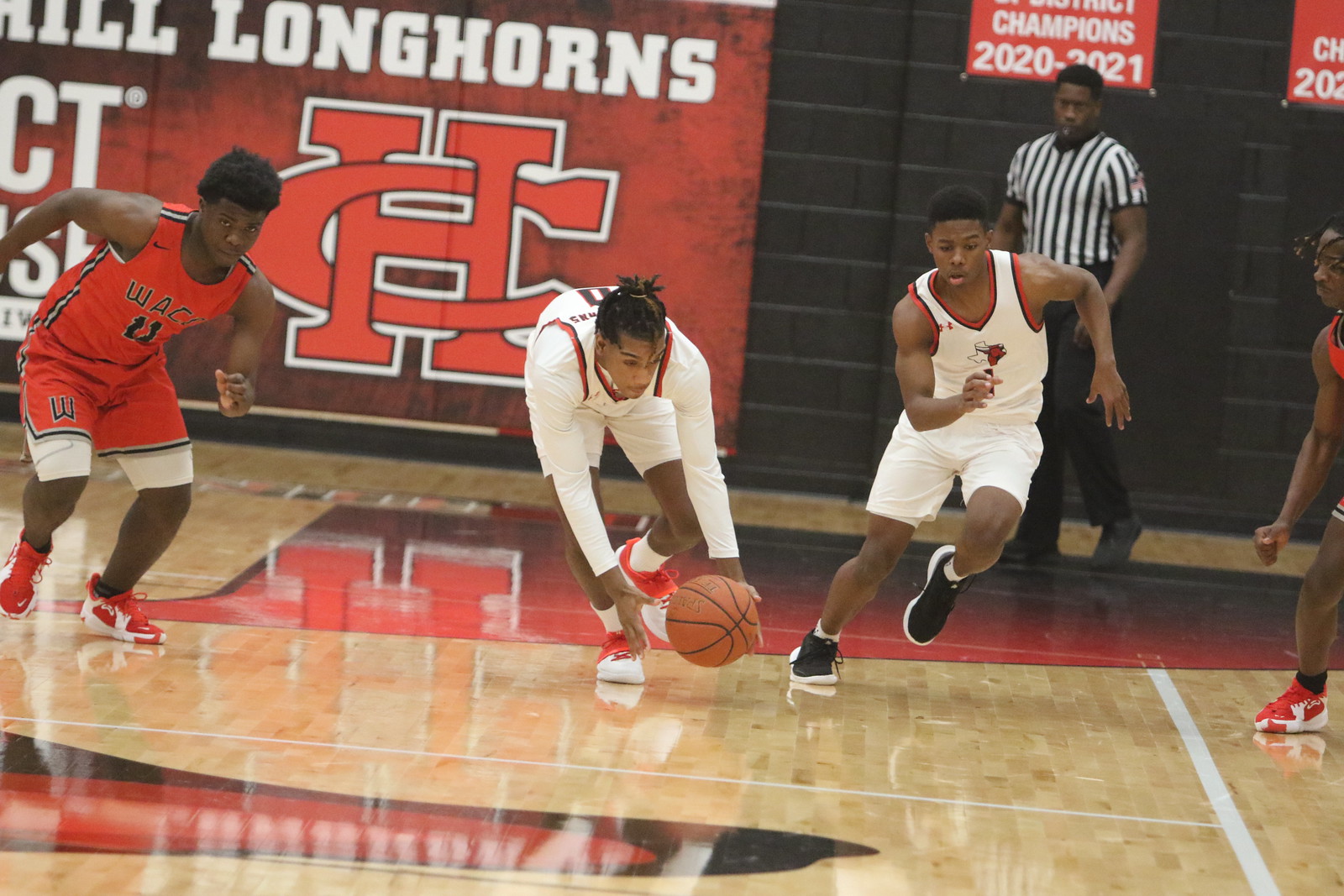The image captures an intense moment of a basketball game being played indoors, featuring African-American players from two teams. The team in white has uniforms with red stripe accents around the arms, and their players sport a combination of long-sleeve compression shirts and sleeveless jerseys. The opposing team is dressed in all-red with white trim on their shorts and red shoes. The central focus is a player in white, diving to catch a ball near the ground, while another player in white runs close by. Two players from the red team are also visible, with one having frizzy black hair. A coach, likely from the white team, and a referee are also present in the background. The gym floor is a shiny beige with red markings. Overhead, banners bearing phrases such as "Champions 2020-2021" and "Hill Longhorns" are displayed prominently, alongside a large one featuring an 'H' intertwined with a 'C', both in red.